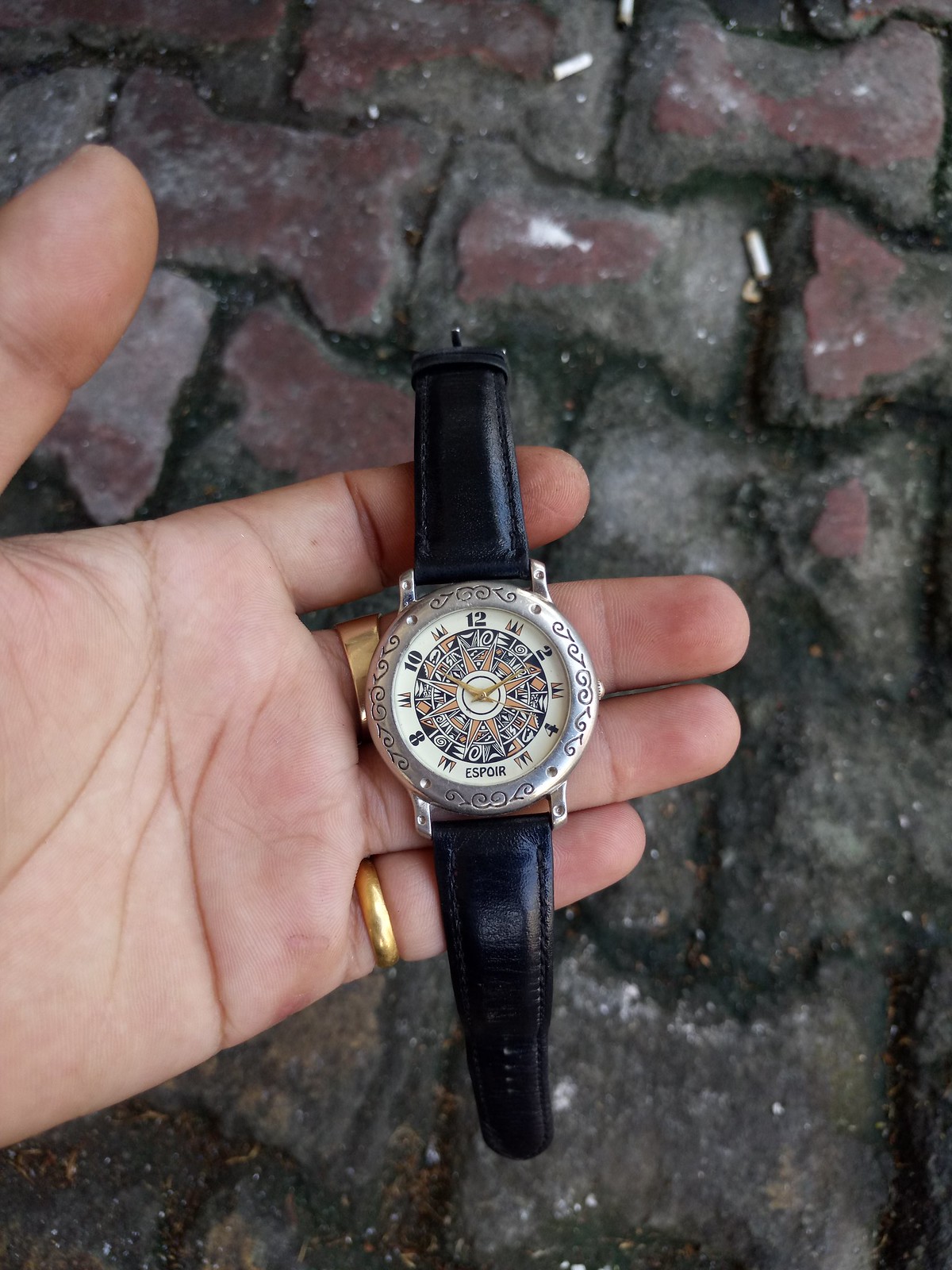This detailed photograph features a unique watch that prominently displays an astrological dial. The watch boasts a double bezel design. The outer bezel is crafted from what appears to be actual silver, adorned with intricate engravings of interesting symbols and signs. Among these engravings are four dots, interspaced with designs that seem to carry astrological significance.

The inner bezel merges seamlessly with the watch's dial, showcasing indicators for the 2, 4, 8, and 10 o'clock positions. Various symbols take the place of numerals for the 1, 3, 5, 7, 9, and 11 o'clock positions, further emphasizing its astrological theme. At the very center of the watch, a sun display evokes the essence of astrology, featuring what seems to be a multipoint star, though the individual symbols are too small to discern clearly.

The watch hands for seconds, minutes, and hours are tinged with gold and orange hues, adding a touch of elegance. The timepiece is secured by a black strap. A hand wearing two gold rings holds the watch, and the background reveals a distant view of gray pavers, subtly completing the scene.